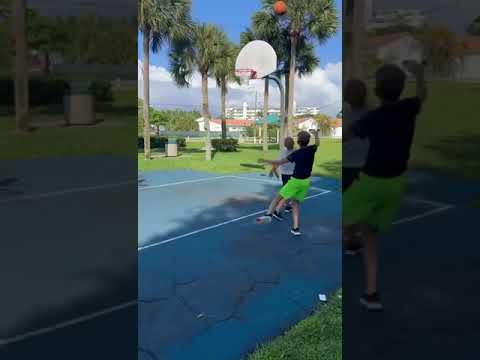In the bright sunshine of a likely Californian day, two young boys are absorbed in a game of basketball on a greenish-toned concrete court. Palm trees sway gently in the background, casting shadows along the edge of the verdant grass surrounding the playing area. Above, the sky is a radiant blue with patches of fluffy clouds. In the distance, there are houses with white walls and orange roofs, and a hint of the ocean shimmering behind, possibly even a ship sailing calmly. 

The boy closest to the camera – dressed in striking neon green shorts and a black T-shirt – has just shot the ball, his left leg raised and arms positioned in the follow-through of his throw. His playmate, clad in a white T-shirt and black shorts, stands nearby, watching intently to see if the shot will be successful. Both boys sport black shoes with white bottoms. Benches and a trash can mark the edges of the court, emphasizing that they are likely in a park setting.